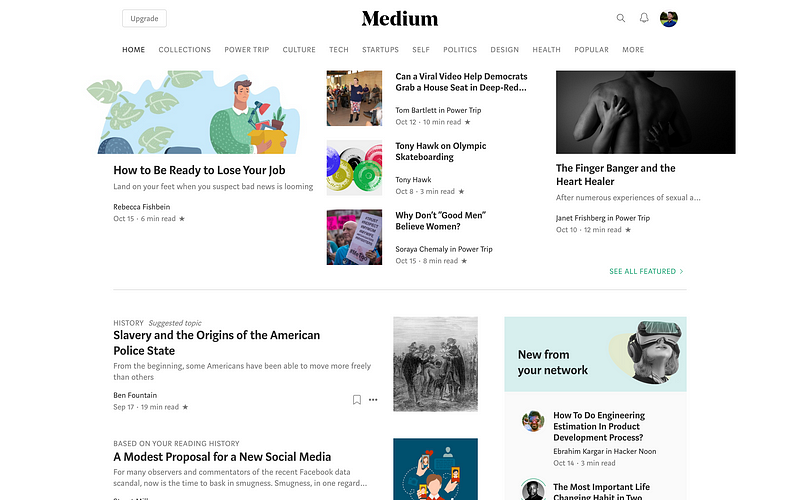**Homepage of Medium: Detailed Layout and Articles**

The homepage of Medium displays a clean and minimalist design with a white background. 

**Header:**
- **Upper Left Corner:** A rectangular button labeled "Upgrade".
- **Center:** The word "Medium" in bold black text.
- **Far Right:** Icons for search (magnifying glass), notifications (bell), and user profile (person icon within a circle).

**Navigation Bar:** Below the main header, the navigation bar lists the following categories in sequence: Home, Collections, Power Trip, Culture, Tech, Startups, Self, Politics, Design, Health, Popular, More.

**Main Content Area:**
1. **Primary Article (Left Side):**
   - Title: "How to Be Ready to Lose Your Job, Land on Your Feet When You Suspect Bad News is Looming"
   - Includes the author's name, publication date, and estimated reading time.

2. **Secondary Articles (Center Column):** Three articles stacked vertically:
   - "Can a Viral Video Help Democrats Grab a House Seat in Deep Red?"
   - "Tony Hawk on Olympic Skateboarding"
   - "Why Don't Good Men Believe Women?"

3. **Featured Article (Far Right):**
   - Displays an image of the back of a man with a woman's arms around him in an embrace.
   - Title: "The Finger Banger and the Heart Healer"

**Additional Articles (Below the Primary Content):**
- Left Side:
  - "Slavery and the Origins of the American Police State"
  - "A Modest Proposal for a New Social Media"

- Right Side:
  - "New From Your Network: How to Do Engineering, Estimation, and Product Development Process"

This layout provides a clear and organized presentation of various articles and categories, facilitating easy navigation and reading for users.